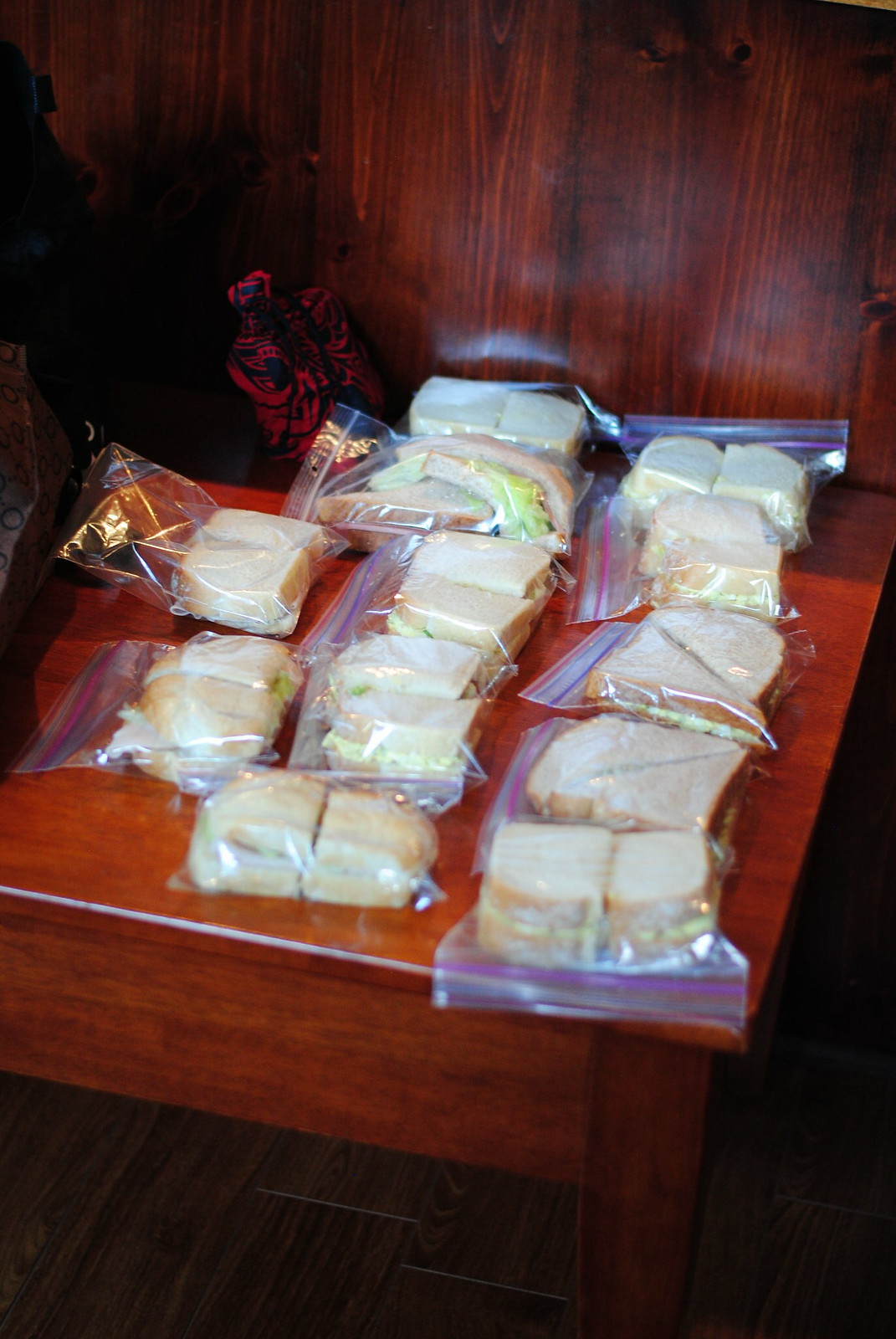The image features a polished, reddish-brown cherry wood table with a darker brown grain, situated against a matching dark cherry wood wall that displays noticeable wood grain lines. The well-lit setting gives a slight glare on the back wall. Sitting atop the table are 12 handmade sandwiches packed in clear, Ziploc-style snack bags with blue, red, or purple zippers at the top. The sandwiches, made with white bread, are cut either vertically or diagonally. In the left corner of the table, there is a dark-colored, uniquely designed bag, although it's difficult to discern specific details due to the shadowy area. The table and sandwiches rest on a brown wood floor, further enhancing the cohesive wooden theme of the scene.